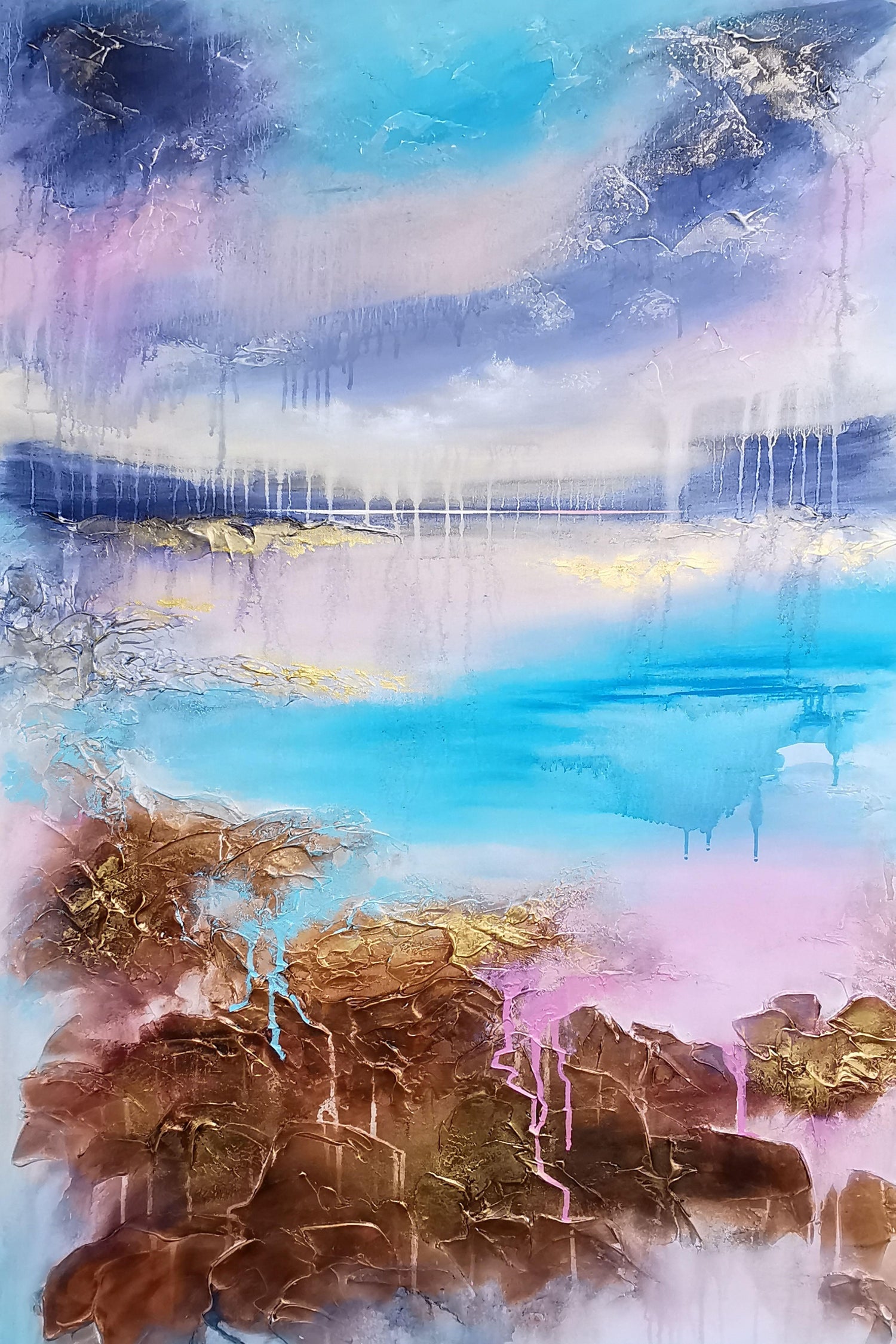This vertically-oriented, abstract art piece, possibly AI-generated, bursts with vibrant colors and intriguing textures. At the top, deep, bold purples blend into rich turquoise, featuring intentional, expressive paint drips. Moving downward, the palette transitions through pinks and whites, with hues that could evoke a sky meeting water. The bottom of the image is dominated by a dynamic mix of coppery browns and golden accents, resembling a rocky shore. The middle section showcases a bright, vivid light blue, contrasted by purples and pinks above. The drip patterns, combined with purposeful lines, create an image that suggests a rocky shore leading out to a distant, mountainous horizon, despite its abstract nature. The textures are heavy and oil-like, especially towards the center, contributing to the overall visual depth and complexity of the painting. The vibrant colors and lack of a distinct pattern make this a compelling and evocative piece.